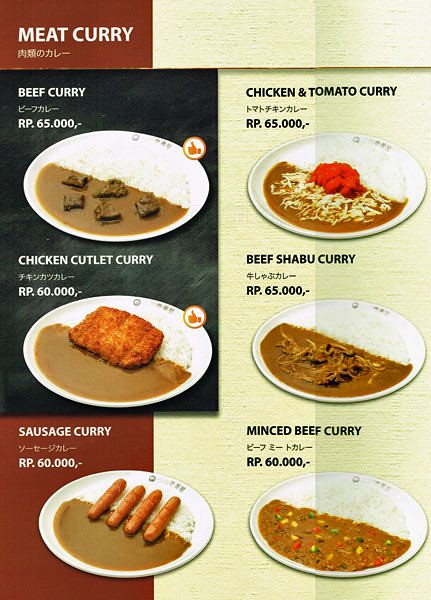The image is a vertical rectangle showcasing a restaurant menu sheet. The right two-thirds is a light gray or tan paper texture, while the left third features a burgundy-red banner running vertically. Centered on this red banner is a black rectangle with white font, listing two dishes: "Beef Curry," followed by Asian characters and priced at RP 65,000, and "Chicken Cutlet Curry," also followed by Asian characters. The Beef Curry is depicted as a white plate half-covered with brown sauce and five pieces of beef over white rice. The Chicken Cutlet Curry shows a white plate divided between brown sauce, white sauce, and a fried chicken piece. At the top left corner of the menu, the text "Meat Curry" is prominent, and below it are six pictorial examples of different dishes including Beef Curry, Chicken and Tomato Curry, Chicken Cutlet Curry, Beef Shabu Curry, Sausage Curry, and Minced Beef Curry, each specified with prices ranging from RP 60,000 to RP 65,000. The entire menu page integrates accent colors such as brown, yellow, black, white, green, and burgundy.